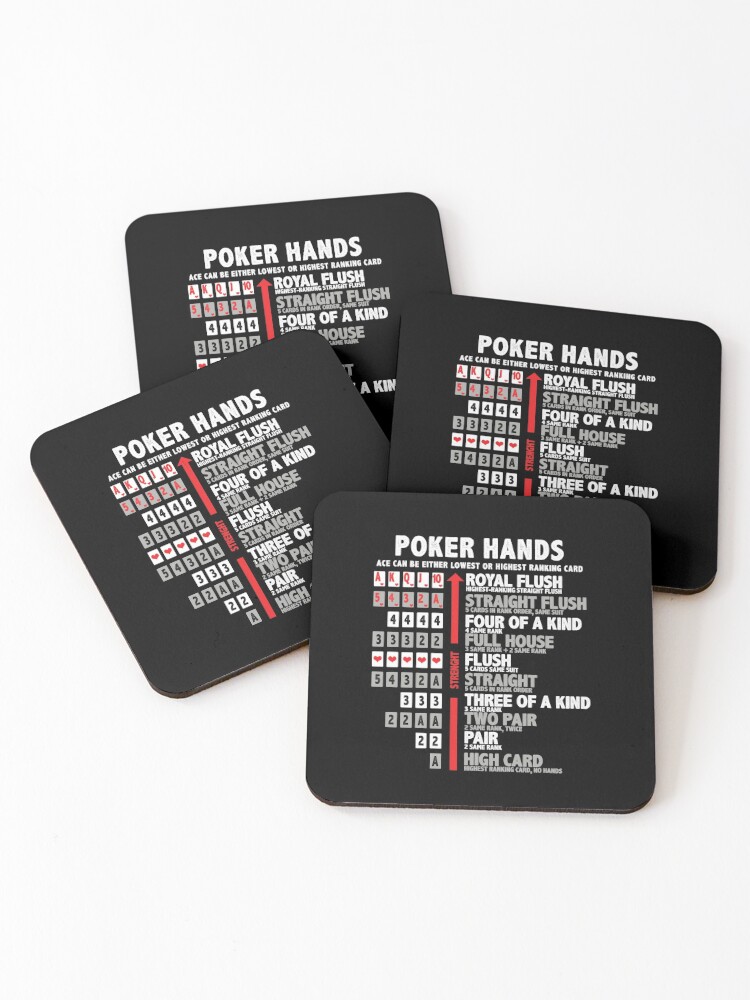The image shows four black coasters with detailed white text outlining poker hand rankings. Each coaster features a red arrow pointing right, where the text lists poker hands in descending order: royal flush, straight flush, four of a kind, full house, flush, straight, three of a kind, two pair, pair, and high card. The text notes that an ace can be either the lowest or highest ranking card. Accompanying the descriptions on the left side of the arrow, the coasters display examples of each hand, such as "A, K, Q, J, 10" for a royal flush, sequences of "5, 4, 3, 2, 8" for other hands, and patterns like "3, 3, 3" or "2, 2" to illustrate different combinations. Essentially, these coasters serve as a handy reference guide for poker players, detailing various possible hands and their rankings.